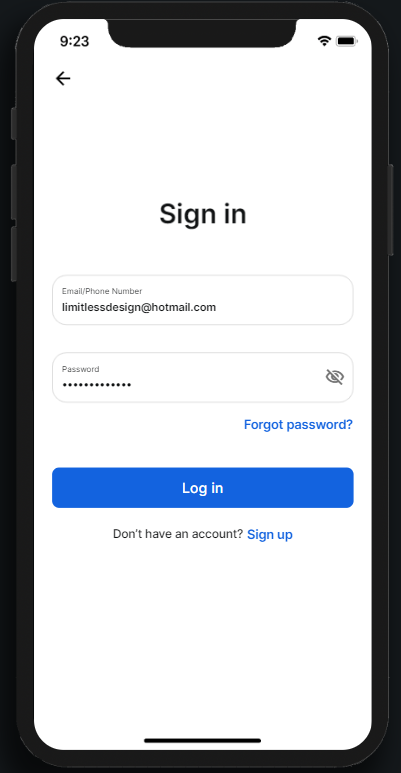This image is a detailed screenshot of a cell phone login screen, framed by a black border with a white background. The time is displayed at the top left corner as 9:23, with icons for wireless signal, Wi-Fi signal, and a fully charged battery on the upper right corner. Below the time, a black left-pointing arrow indicates a back navigation option. 

Prominently centered at the top is the title "Sign In." Below, the login form consists of two input fields. The first box is labeled "Email / Phone Number" with the entered email "limitlessdesign@hotmail.com." The second box is titled "Password," protected by 13 black dots to obscure the entered password, with the eye icon grayed out indicating the option to show the password is currently disabled. 

Adjacent to the password box, a blue "Forgot Password?" hyperlink is available for password recovery. Further below, there's a blue rectangular button with the word "Login" in white, serving as the primary action button. At the bottom, an invitation "Don't have an account? Sign up" is displayed, with "Sign up" as a clickable blue hyperlink directing users to the account creation page. There is no additional text present.